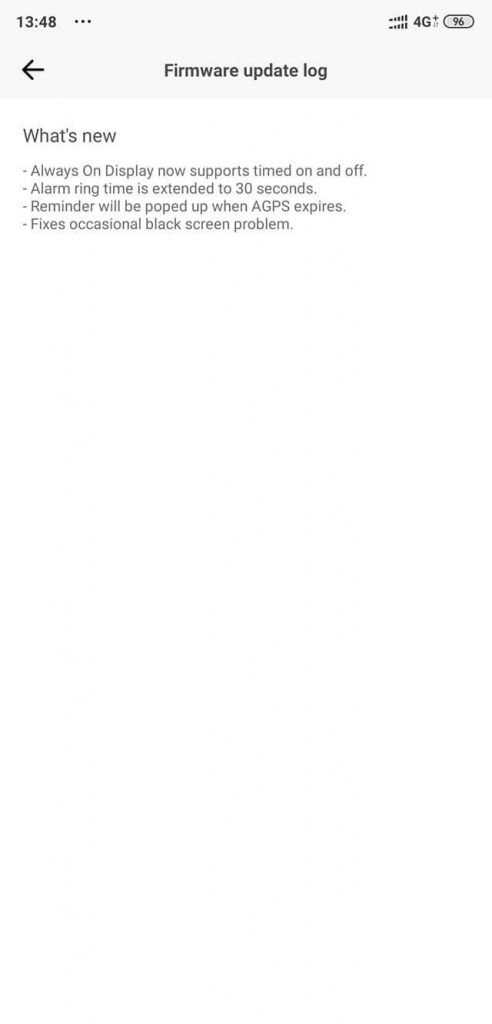**Caption:**

The image depicts an interface screen with a very light gray background stretching across the top portion of the display, resembling a rectangular bar. Centered in this bar, the time is displayed in black as "13:48" (or 1:48 PM). Adjacent to the time, three black circles are aligned horizontally.

Additionally, the interface features an interesting display of what appears to be dual reception signals, stacked one above the other, forming a series of rectangles indicating full reception and battery charge. To the right of this, "4G+" is prominently displayed.

Adjacent to the signal indicators, a light gray oval outlined in a darker gray showcases the number "96", likely representing the battery percentage.

On the following row, a black arrow pointing to the left is displayed next to the text "Firmware Update Log" in bold black font. Below this header, the background turns white, with the section titled "What's New" in black font. A list of updates follows in a smaller font:

- Always-on display now supports time on and time off.
- Alarm ring time is extended to 30 seconds.
- Reminder will pop up when AGPS expires.
- Fixes occasional black screen problem.

The detailed layout and structured presentation provide a comprehensive and easy-to-follow update log for users.